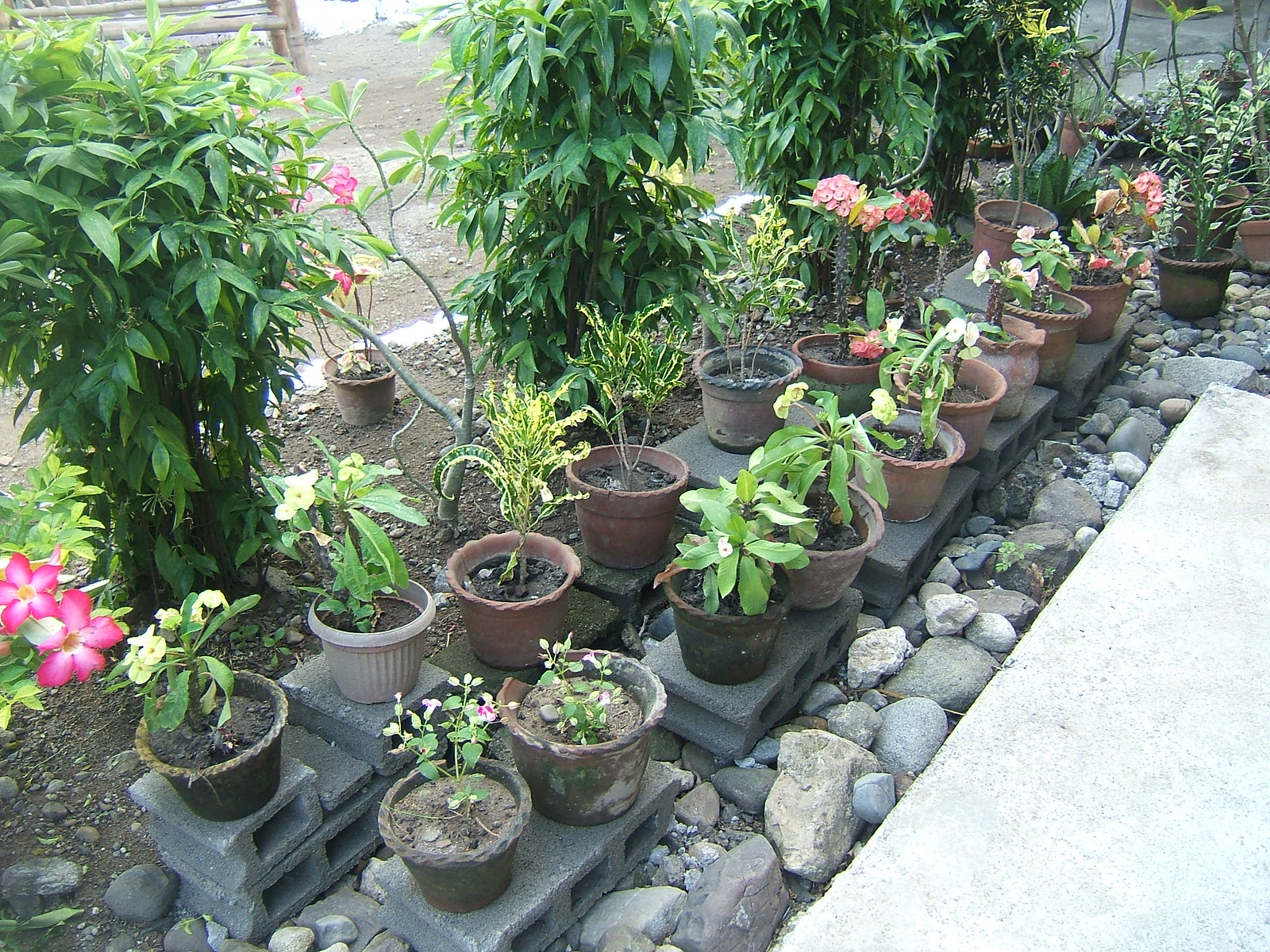The photograph is an outdoor garden scene taken on a bright, potentially cloudy day with a cyan or blue tint and low saturation. It displays two rows of potted plants arranged diagonally from the bottom left to the top right, sitting on gray cinder blocks. Each row contains approximately eight pots, with some cinder blocks holding two pots and others just one. The pots are primarily orange terracotta, with a few white and brown ones mixed in. The plants vary, including both green leafy types and those with flowering blooms in pink, yellow, orange, and red. Toward the back in the top right, some plants have vibrant pink and white flowers. 

The left side of the image features a wall with taller green foliage, and dirt is visible in the background. On the right side at the bottom, there is a rock garden composed of fairly large gray and off-white stones next to a white cement or sidewalk area. Additionally, behind the rows of potted plants, there are four large bushes with bright green leaves extending down their length. In the distance, tall trees and a stone gravel pathway or driveway suggest the boundary of the garden.